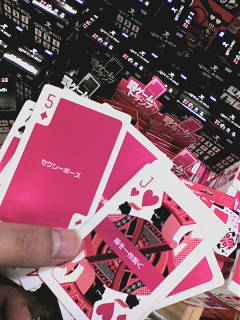A tan hand is prominently displayed, holding a fan of hot pink playing cards. Among the cards held, visible are a Jack of Hearts, a Five of Diamonds, and a partially obscured Seven of Clubs. The Five of Diamonds features a minimalist design with a solid color block background and text in an Asian language. The Jack of Hearts, while retaining its traditional form, is uniquely colored in black, hot pink, and hints of red. The face of the Jack is entirely black, with pink hair and a hat, accented further by red and black in the clothing. Behind the hand, multiple boxes of the same set of playing cards are visible, suggesting a collection or display.